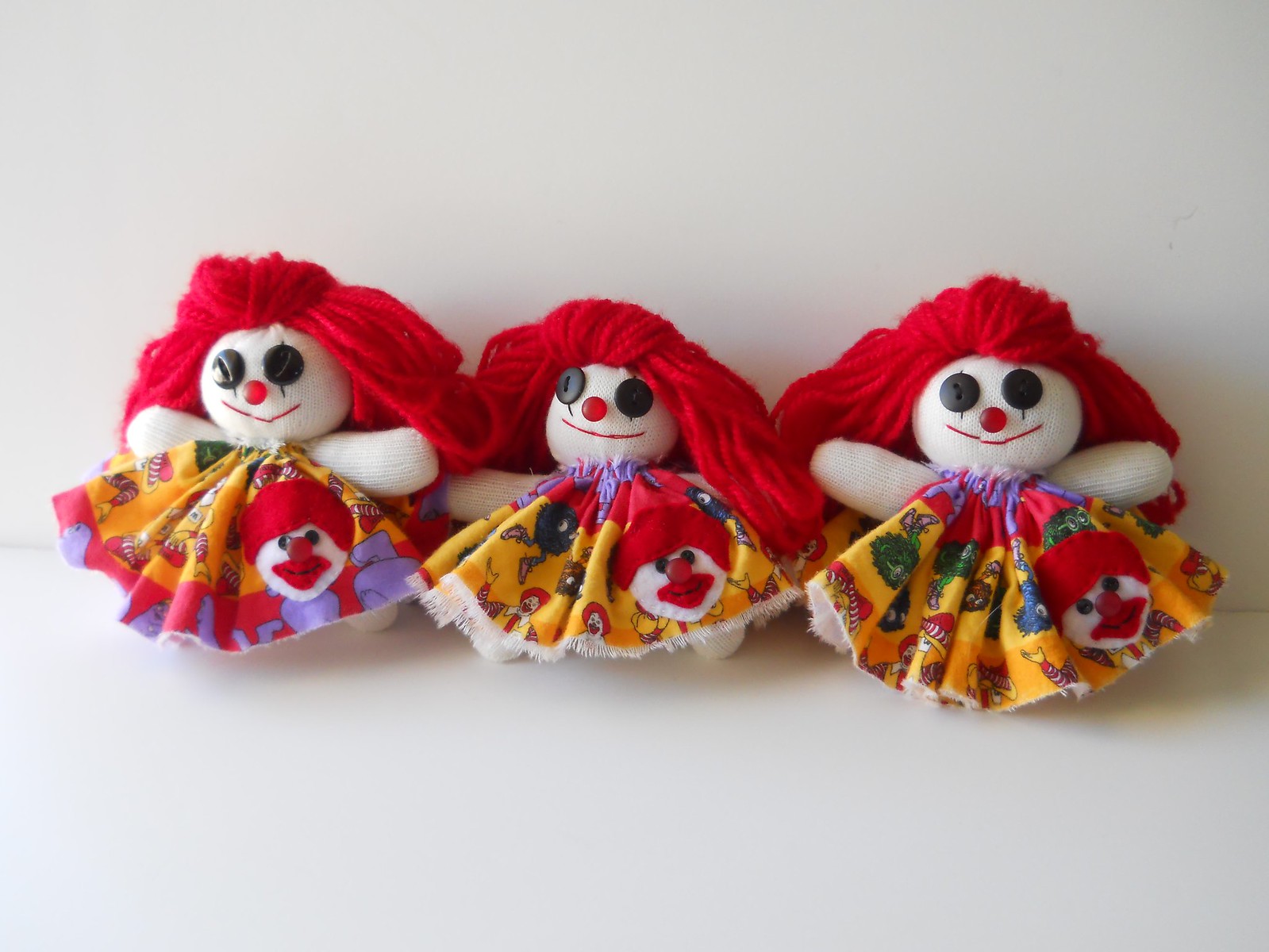This is a horizontal image of three homemade Raggedy Ann-type dolls arranged side by side at the center, photographed against a plain white background. Each doll features distinctive long, red yarn hair, large black button eyes, a smaller red button nose, and a red embroidered smile on their round, white, stuffed faces. Their dresses share a common design and color scheme consisting of red, purple, white, and green. A prominent detail on the right-hand side of each dress is a patch featuring a clown face resembling Ronald McDonald, with red felt hair, a white felt face, small black felt eyes, a red button nose identical to that of the dolls, and black felt lips. The overall imagery and arrangement create a charming, cohesive presentation of these handcrafted, nostalgic dolls.